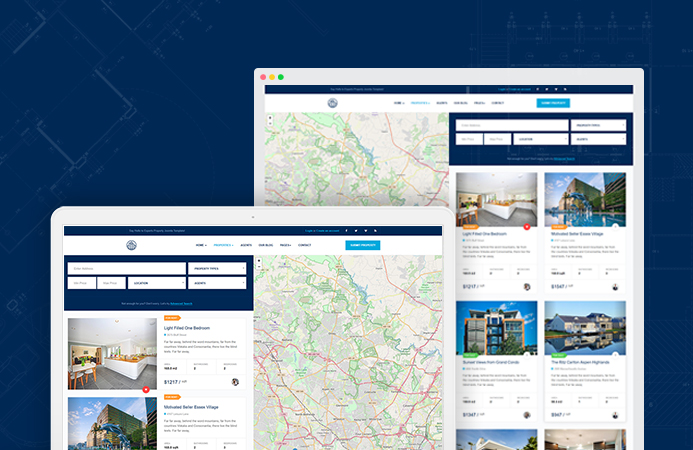A detailed descriptive caption of the screenshot:

"The image appears to be a screenshot of a PC or tablet displaying a lodging search website. The website boasts a medium dark blue background adorned with faint, neat, architectural-style line drawings that add a sophisticated flair without overwhelming the viewer. The webpage layout consists of two nearly identical sections, partially superimposed over each other, both displaying search results for lodging options in the same location.

The lower section, positioned slightly to the left, features truncated elements at the bottom, including two small thumbnails showcasing different lodging spots. To the right side of this section, there is a faint blue and white map adorned with standard red markers indicating various locations.

The second section, partially obscured by the aforementioned lower section, is positioned towards the upper right corner and contains a more extensive collection of lodging thumbnails—at least six are visible. One of these thumbnails distinctly represents a private house, suggesting that the listings could include rental properties in addition to traditional vacation lodging.

Both sections share a consistent design in the upper left corner, presenting the essential search text boxes typically employed for inputting location and lodging criteria. Although the text within the thumbnails is too small and blurry to read, the overall layout and elements unmistakably classify this site as a platform for searching and browsing lodging or rental properties."